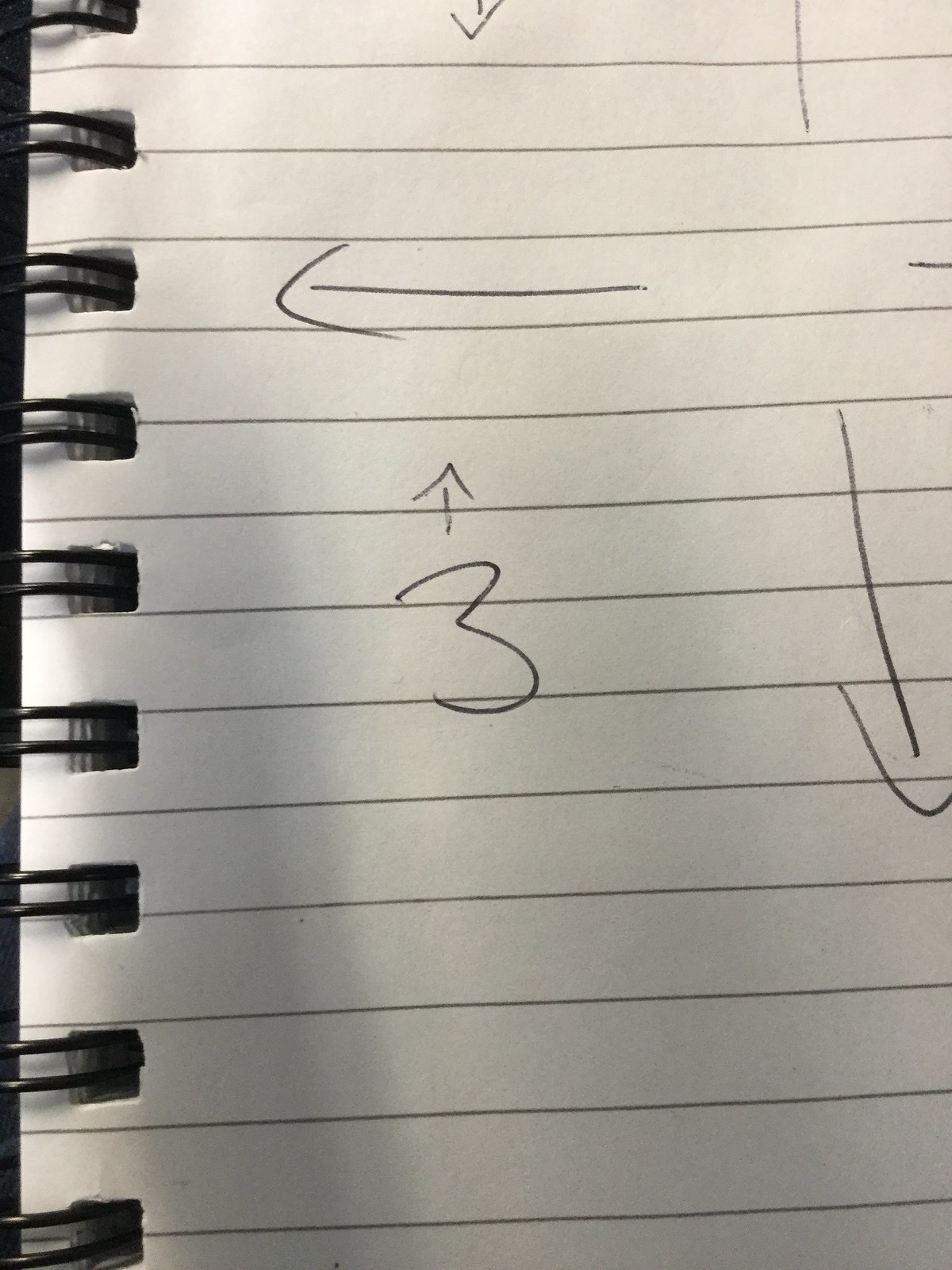The image captures a small section of a spiral-bound, lined notebook. In this fragment, the spiral binding is visible in eight places. The lighting creates the shadow of a couple of fingers, suggesting the photo was taken while someone held or manipulated the notebook. On the notebook’s lined paper, various pen marks include two arrows—one pointing downwards and another pointing to the left. Nestled between these arrows is the number “3” with a tiny arrow pointing up. Additionally, there are faint traces of other arrows—one partially visible above the left-pointing arrow, and two lines suggesting the presence of more arrows pointing upwards and to the right, hinting at a possibly complex diagram or list trailing off the frame. The scene feels like a snapshot of someone's hand-drawn calculations or notes, the specifics of which remain unclear.